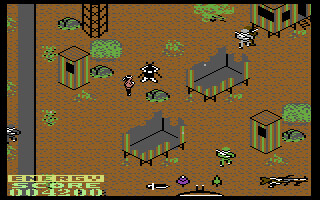The image is a heavily pixelated color screenshot from an early, two-dimensional video game, making it difficult to discern all details. The scene is set on a brown, dirt-colored field dotted with green bushes. There are various characters visible, including a bare-chested figure with a white headband and several small robotic or animal-like characters. These characters appear to be interacting with one another on this landscape. The game includes several structures, some resembling damaged huts on stilts and buildings with wooden roofs and small square black windows. A wire structure tower can be seen in the upper left-hand corner, and a gray border or fence is visible on the left side of the playing area. In the bottom left-hand corner of the screen, the text "ENERGY SCORE 004200" is displayed, with the word "ENERGY" highlighted in yellow, suggesting an important gameplay element.